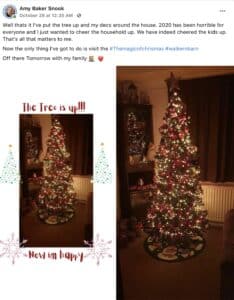The image comprises a faint gray line at the top, beneath which lies a circle containing a picture, accompanied by tiny black text to its right. Below this is a small paragraph in black. A halfway-down black line separates text to the right written in blue, followed by additional black letters and two symbols beneath it—a red heart and an indistinguishable shape. The image also features two smaller pictures below: the first depicting a room with potential Christmas decorations, such as a tree and possibly a cabinet window, adorned with red text above and below it. Surrounding these pictures are green dot-shaped Christmas trees and pale red snowflakes. The larger image of the Christmas tree reveals curtains in the background and a cabinet on the left-hand side.